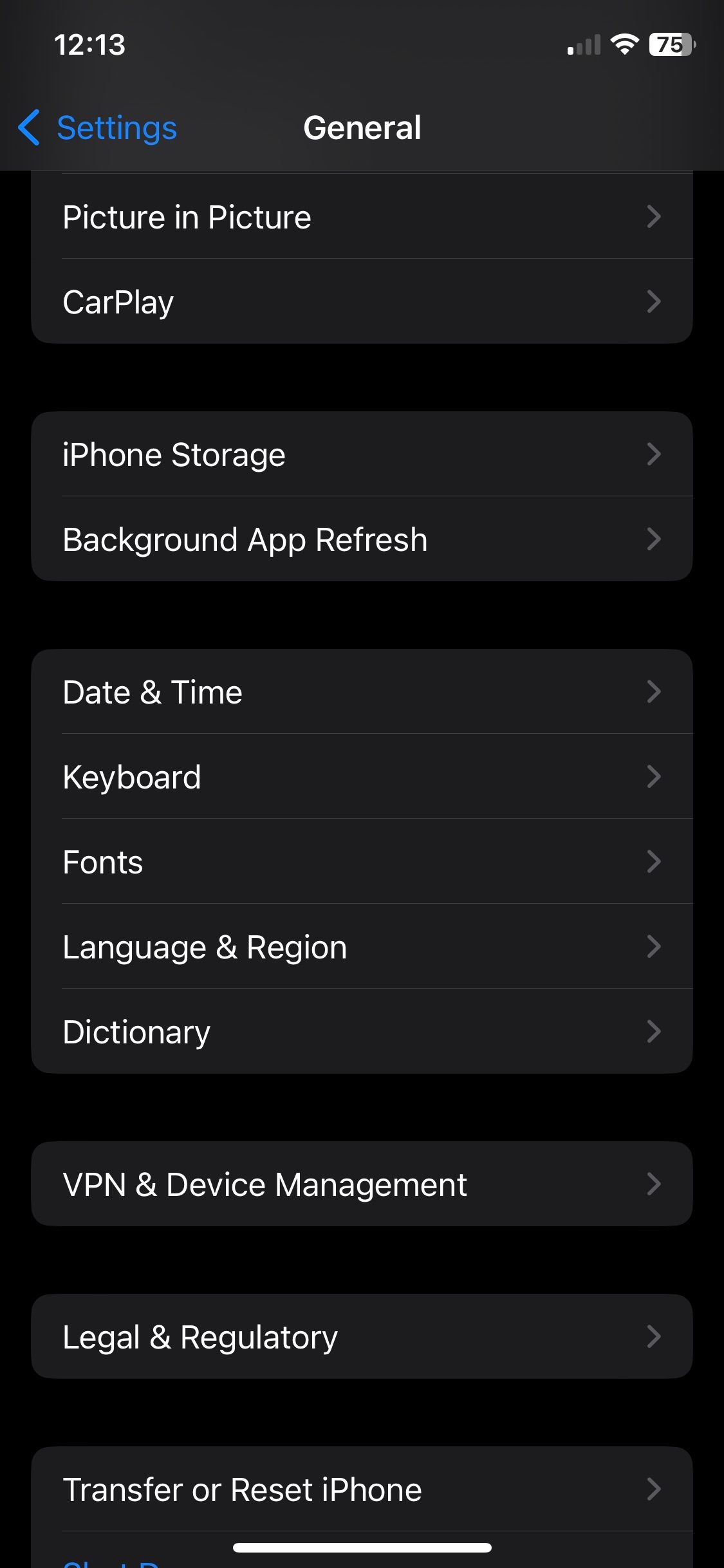This is a detailed screenshot from a smartphone. The background is black with dark gray text boxes. In the upper left corner, the time reads "12:13." On the right side of the screen, there is one bar of cell service, Wi-Fi connectivity, and a 75% battery level indicator. 

Below the status bar, the interface displays navigational elements. A blue right-facing arrow next to the word "Settings" in blue and "General" in white signifies the current menu. The subsequent sections are listed with right-facing arrows on the right side of each entry. The background alternates between light and dark gray, and the text is all in white. 

The menu options are as follows: "Picture in Picture," "CarPlay," "iPhone Storage," "Background App Refresh," "Date & Time," "Keyboard," "Fonts," "Language & Region," "Dictionary," "VPN & Device Management," "Legal & Regulatory," and "Transfer or Reset iPhone." 

At the bottom center of the screen, there is a prominent thick white line.